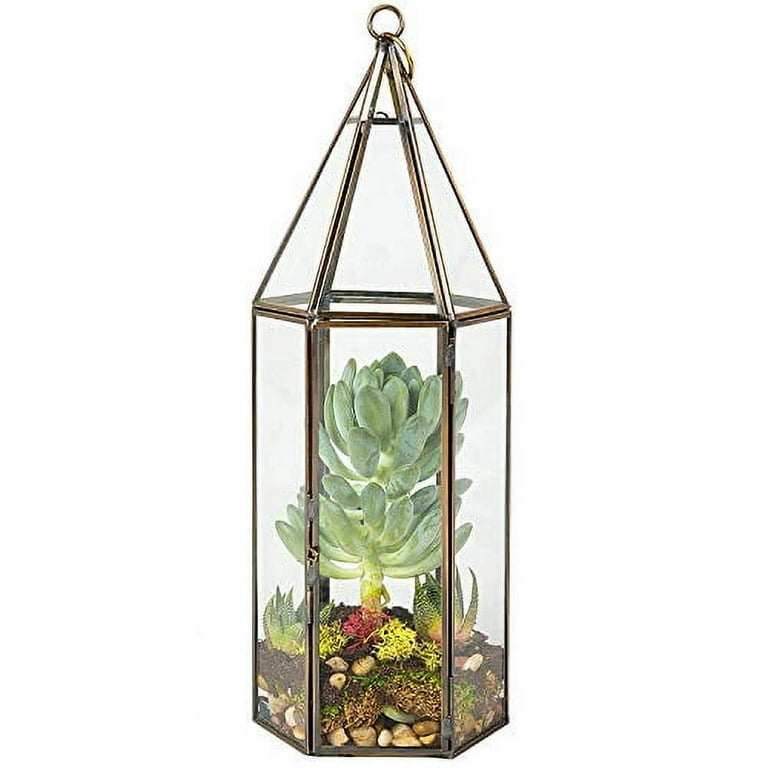This full-color photograph depicts a meticulously staged terrarium housed within a hexagonal glass and brass lantern. The lantern, featuring vertical and horizontal brass supports, tapers into a pyramid-like shape at the top. An o-ring at its peak allows for hanging. Inside, the scene is composed of layered, multi-colored rocks, brown soil, and patches of moss. Dominating the arrangement is a central green cactus-like succulent with thick, artichoke-reminiscent leaves, surrounded by several smaller succulent plants. The crisp white background emphasizes the vibrant details and textures within the lantern, making the entire setup appear as though it is floating on the canvas of the computer screen.